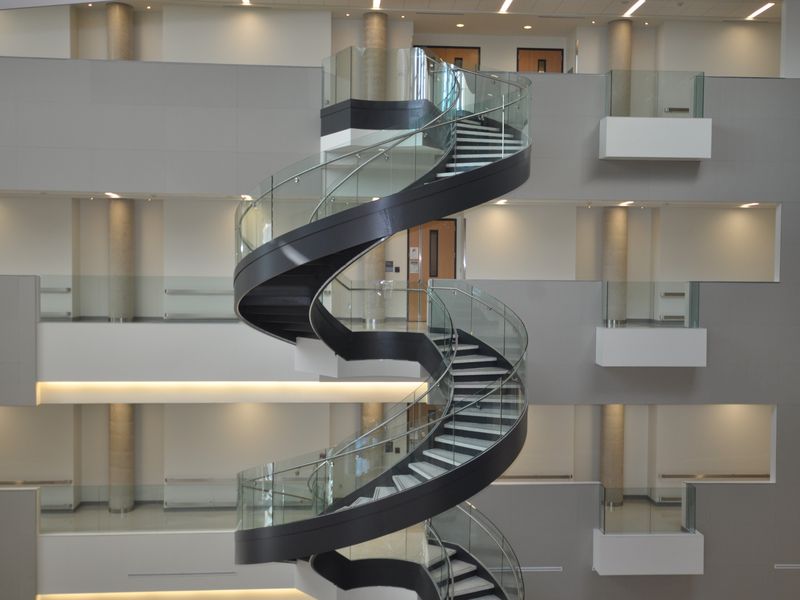This photograph captures the interior of a multi-story office building featuring a striking spiral staircase that extends through three levels. The central staircase is a combination of silver and black steps with a transparent plastic guardrail, offering a modern and sleek design. Each level is connected by this winding staircase, and the floors are covered in elegant gray, marble-like material. The white walls and tan columns on each floor contrast sharply with the architectural beauty of the staircase. The top level displays two brown wooden doors, while the middle level has one visible wooden door. Lighting is strategically placed throughout, with small, narrow lights spaced approximately every 5-10 feet across the ceiling, illuminating the floors and enhancing the brightness of the space. Adding to the ambiance, the staircase area includes glass balustrades, allowing for clear views across the different levels, giving a sense of openness and connectivity throughout the building.